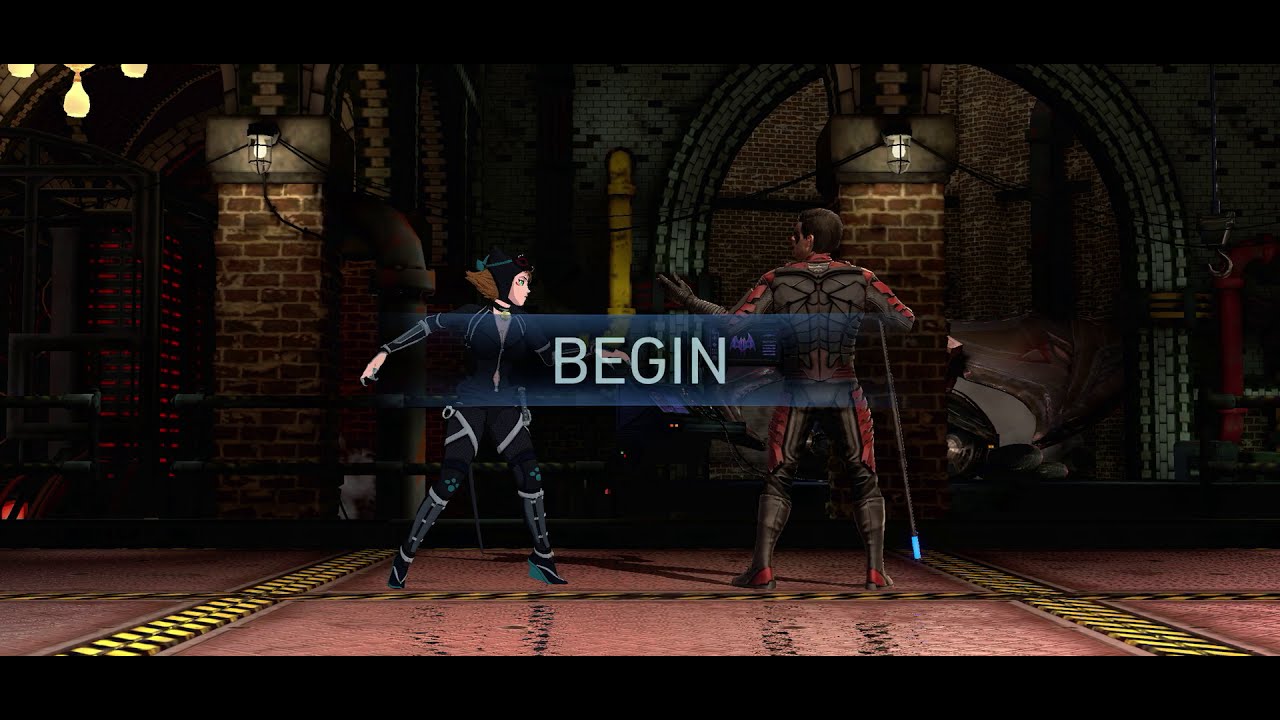The image is a detailed screenshot of a fighting game, featuring two characters in an intense standoff. The scene, reminiscent of Mortal Kombat, showcases a 1v1 fight with the word "BEGIN" prominently displayed in translucent white letters at the center. On the right, a male character resembling a black-suited superhero holds a cane, his attire a mix of black, red, and brown. On the left, a female character in a dark blue tech suit, equipped with goggles, faces her opponent. Notably, her art style is more anime-influenced, contrasting with the more realistic design of her male counterpart.

They are positioned in what appears to be an underground arena with a setting evocative of a secret lab or an abandoned subway. The floor they stand on is terracotta-colored pavers, marked with yellow and black lines running from the foreground to the back of the scene. The background is a dark, dungeon-like environment with red and white brick walls, archways, barred sections, and industrial light fixtures resembling cages hanging from the ceiling. The atmosphere is gritty and suspenseful, perfectly setting the stage for an epic fight.